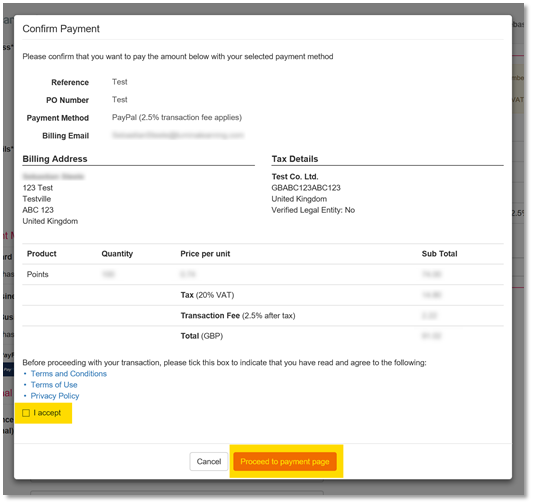Caption: 

The image displays a payment confirmation screen. At the top left corner, it prominently reads "Confirm Payment." The prompt requests the user to confirm their intent to pay the specified amount using their selected payment method. Under "payment reference method," it is listed as "PayPal," with a parenthetical note indicating that a 2.5% transaction fee applies. The user's billing email is shown but blurred for privacy. The billing address is presented with the first line obscured, followed by "123 Test Test Avenue, ABC 123, United Kingdom."

Under "tax details," it lists "Test Company LTD, LTB," with the VAT number "GB ABC 123 ABC 123," and mentions that the legal entity is "not verified."

A table summarizes the purchase, displaying labels for "Product," "Quantity," "Price per Unit," and "Subtotal." The first product line, as well as lines for "Points" and "Transaction fee 2.5% after-tax," have their details blurred. The "Tax at 20% VAT" line is also present, with details hidden. Lastly, the table concludes with the "Total (GBP)" line, which is similarly blurred for obscurity.